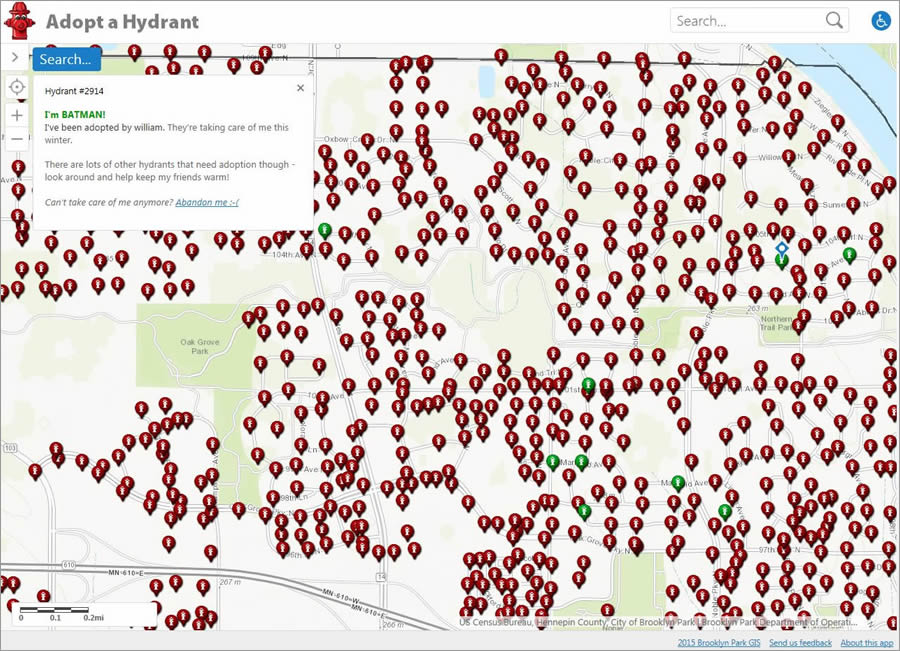The image depicts an interactive computer screen showcasing a detailed map titled "Adopt a Hydrant." At the top left, the map features a red fire hydrant symbol next to the title, with a search bar and accessibility icons on the far right. The map highlights the locations of numerous fire hydrants across the city. Notably, hydrant number 2914 is flagged with a green label that reads, "I'm Batman! I've been adopted by William, they're taking care of me this winter." This hydrant, along with several others, stands out in green to indicate adoption status. Numerous red pins mark the other hydrants still available for adoption, encouraging users to "look around and help keep my friends warm." Clicking on these pins provides further details about each hydrant. The map includes the parks Oak Grove Park and Northern Trail Park, though street names are barely visible. At the bottom right, credits read "U.S. Census Bureau, Henn-Benden County, City of Brooklyn Park, Brooklyn Park Department of Operations" and "2015 Brooklyn Park GIS," with hyperlinks for user feedback. The far left corner of the map features a legend for the map's scale, enhancing user navigation.